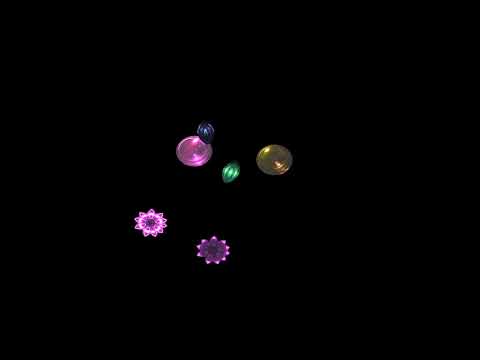The image features five jewelry-like objects set against a stark black background, enhancing their illuminated appearance. At the top, there's a round pink piece that stands out due to its bright, almost self-illuminating quality. To the right of it, a gold circular piece adds a contrasting elegance. Between these two, a highly illuminated green object captures attention with its vibrant hue. Below them are two star-like pieces of jewelry, both pink and prominently illuminated, particularly the one on the left, which seems to glow on its own. The objects, varying in shapes such as ovals and circles with intricate designs, including spokes, create a visually striking composition. The solid black background further accentuates the vivid colors: shades of pink, purple, green, yellow, and blue, making the objects appear almost as if they are floating or part of a digital design, enhancing their decorative allure.